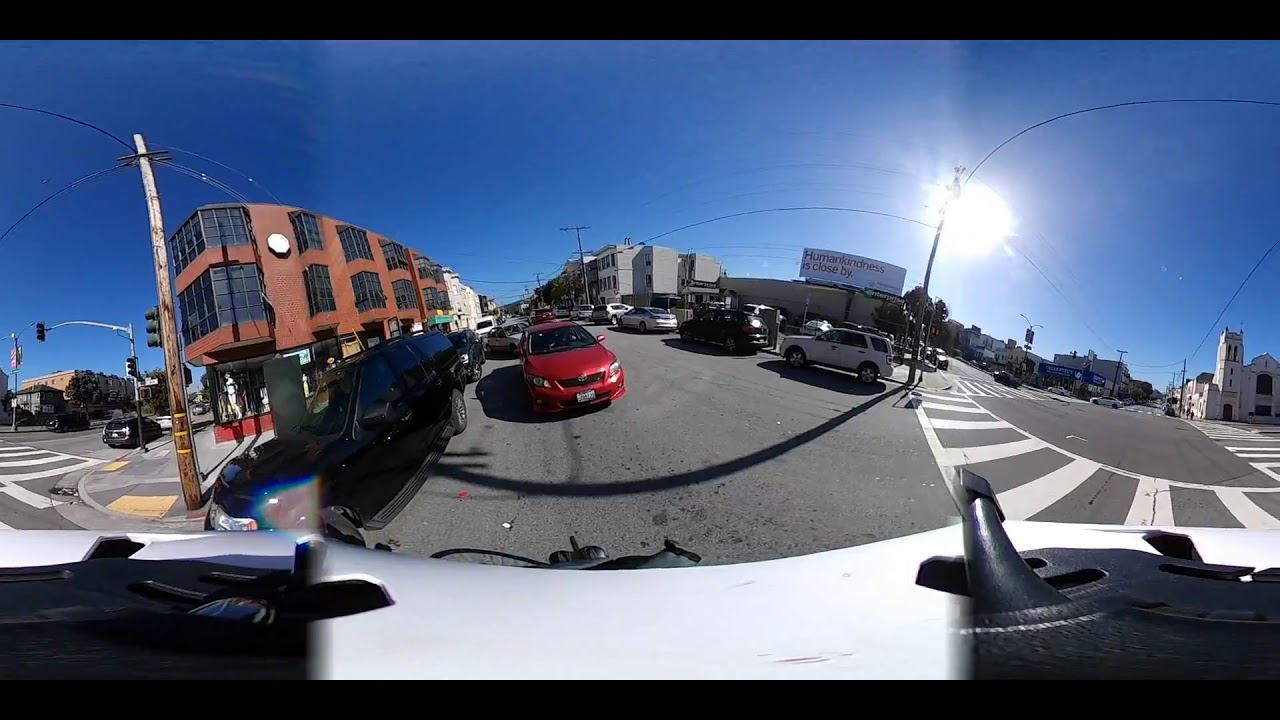A brilliantly blue sky stretches across the top of a distorted wide-angle image, capturing an expansive city street scene from the perspective of a car, as buildings flank both sides. The sun, a white ball, shines brightly from the upper right, casting light over the entire scene. Directly ahead, the street bends and curves in an unusual, almost panoramic fashion, creating a surreal, oval-shaped distortion. Cars, both coming towards and moving away from the viewer, populate the road along with several visible crosswalks, especially prominent on the right where they curve around the street corner. The edges of the image reveal the ends of adjacent streets, furthering the sense of a wide, encompassing view. Traffic lights, power lines, and a variety of colors including black, blue, white, gray, brown, red, and yellow add vivid detail. The scene is bathed in daytime light, making the asphalt, the central street, and surrounding structures clearly visible.